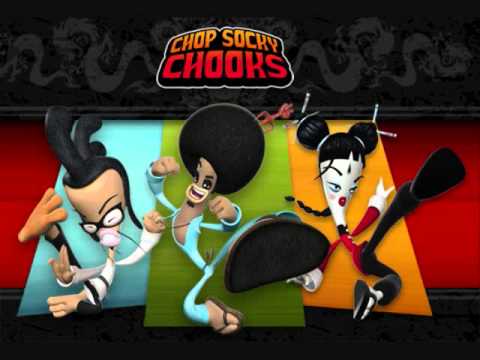The image is a promotional visual for "Chop Socky Chooks," possibly an animated series or video game, characterized by a bold cartoon style. The background is black with subtle, gray-toned dragons exhaling fire at the top, creating a dynamic and intense atmosphere. The title "Chop Socky Chooks" is prominently displayed in vivid yellow and red letters. 

Below the title are three characters, each striking martial arts poses. On the left, a character is dressed in a traditional white gi with black glasses and striking, spiked black hair. The character on the right is adorned with white geisha-style makeup, sporting two hair buns secured with chopsticks, and wearing a red jacket. The central character has a darker skin tone, an afro hairstyle, and is outfitted in a blue bodysuit. 

The characters' exaggerated features and attire might be perceived as racially insensitive, resembling caricatures that perpetuate stereotypes. Their visual design, combined with martial arts themes, hints at a possibly contentious representation of cultural elements.